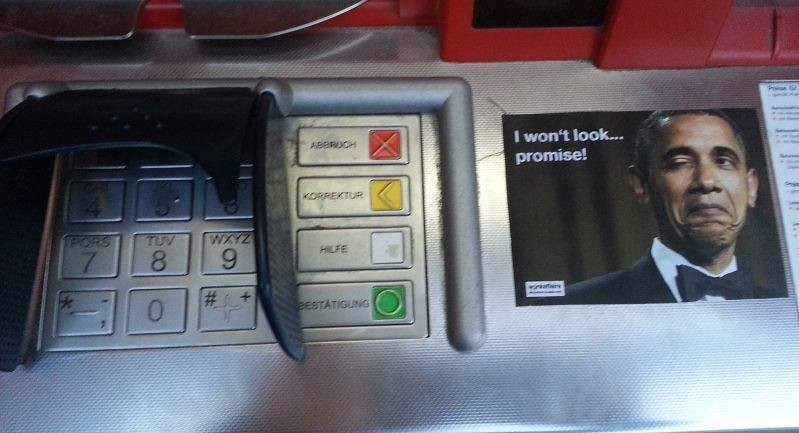The image depicts a metal ATM with a shielded keypad on the left side, featuring numeric dials (1-9, 0), a star (*), and a pound (#) key. The keypad includes colored buttons: red, yellow, white, and green, aligned vertically. To the right of the keypad, a sticker of Barack Obama in a tuxedo with a black bow tie is affixed. Obama is winking and accompanied by the text, "I won't look, promise," suggesting a playful yet sarcastic commentary on surveillance practices. Above the ATM, a red area likely indicates where money is dispensed. The photo, possibly taken in a mall, focuses on the contrast between the secure, functional design of the ATM and the humorous sticker.